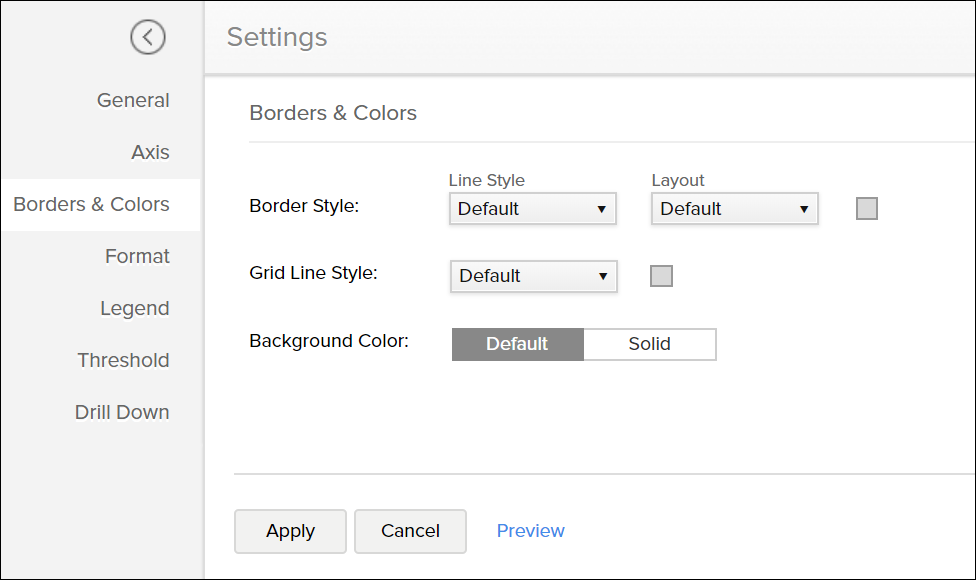The image displays a settings page characterized by a structured layout and a palette of grey and white tones. 

At the top of the page, there is a light grey box with the word "Settings" prominently displayed. Below this header, the section title "Borders" appears in a darker grey font, followed by a thin dividing line. 

Within the Borders section, there are three sub-options:

1. **Border Style**: This includes two dropdown boxes. The first dropdown is labeled "Line Style" and is currently set to "Default." The second dropdown, labeled "Layout," is also set to "Default." An empty text box is positioned next to these dropdowns.
2. **Grid Line Style**: Displayed below the Border Style, this dropdown is similarly set to "Default," and it is accompanied by an empty text box.
3. **Background Color**: This option provides two buttons for selection. The left button, grey in color, is labeled "Default," whereas the right button, white in color, is labeled "Solid."

On the left side of the page, there is a navigation pane within a white and grey box. This pane includes an arrow at the top pointing left and a vertical list of navigation items. The list includes the following options, each represented in plain text: General, Axis, Borders and Colors (highlighted in white), Format, Legend, Threshold, and Drill Down.

At the bottom of the page, there are two functional buttons: "Apply" and "Cancel," with "Apply" on the left and "Cancel" on the right. Additionally, a "Preview" link appears in blue text, presumably offering a way to review the settings before applying them.